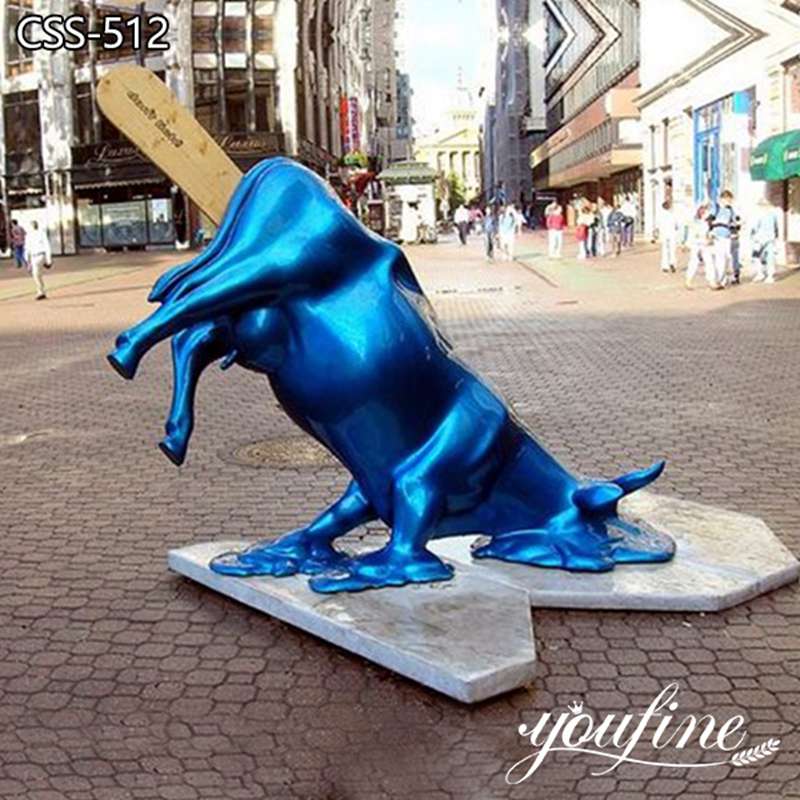The photograph captures a bustling city square, potentially in a European or Latin American country, adorned with an eccentric modern art sculpture. This centerpiece features a bright blue cow seemingly melting into the brown cobblestone sidewalk and a thin gray concrete slab. The cow's face and front legs appear to be dissolving into the slab, with blue puddles enhancing the melting illusion. Its hindquarters, elevated and defying normality, have a brown popsicle stick-like element protruding from them. On the lower part of the image, the text "YOUFINE" is prominently displayed, underlined by a piece of wheat. People meander through the square, bordered by buildings of various colors. In the top left corner, the alphanumeric code CSS-512 is visible. Behind the scene, tall skyscrapers frame a light blue sky, while a stately government building with pillars is discernible in the distant background.